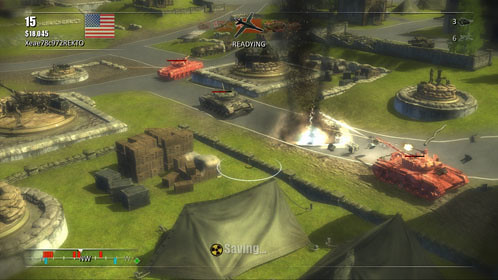The image is a vivid screenshot from a video game, reminiscent of Call of Duty or Warzone, displaying a dramatic action sequence. Dominating the right side, a red tank with a health bar above its cabin is firing, causing an explosion that sends black smoke billowing into the air. A green tank with about 60% health is positioned slightly to the left of center, aligned with another nearly full-health red tank above it. All the action unfolds on a gray paved road surrounded by lush green grass. The battlefield features scattered, half-destroyed monuments, possibly gravestones, and various objects including circular forts, craters, and piles of bricks and boxes. In the upper-left corner, an American flag waves beside the number 15, followed by some unreadable writing. The bottom left showcases a compass navigation tool, while the center bottom displays the word "Saving" next to a nuclear symbol with three spinning black wheels. A red banner at the top center indicates "Readying," accompanied by an image of a jet. Additional details include small numbers 3 and 6 on the right and a green tent set up amidst the chaos.